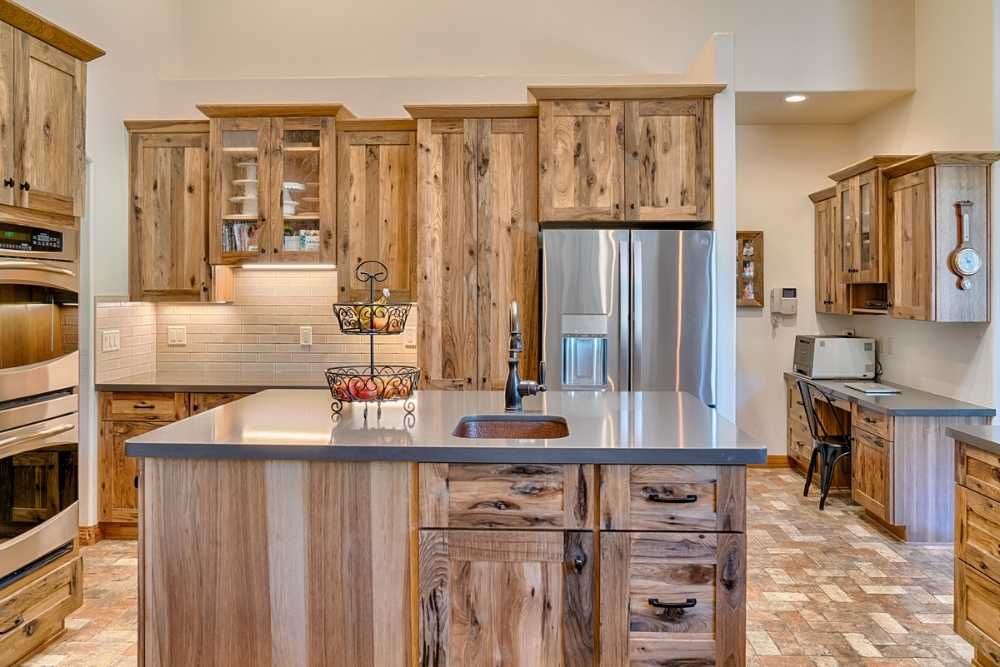This full-color, square photograph captures a beautifully designed, modern kitchen featuring elements of hardwood and stainless steel. The focal point is a central island with a sleek gray marble countertop and a prominently positioned sink with a black faucet. On the island, there's a two-tier metal fruit stand holding various fruits. The base of the island consists of hardwood with four drawers.

The surrounding floor is a multi-shade brown hardwood, adding warmth to the space. Directly behind the island stands a stainless steel refrigerator, with brown wooden cabinets overhead and to the left. To the left of the refrigerator, there's a countertop matching the island's gray marble surface, supplemented by additional cabinets below.

The left side of the kitchen reveals a set of two stainless steel ovens with transparent windows, complemented by wooden cabinets both above and below. On the right, a functional home office space is integrated into the kitchen design, featuring overhead cabinets, a desk with a printer, and a section suitable for a chair.

Adding to the room’s charming utility is a window on the right-hand side, allowing natural light to filter through and blend seamlessly with the warm indoor lighting. A wall-mounted clock provides a practical touch to the kitchen's cohesive and elegant design.